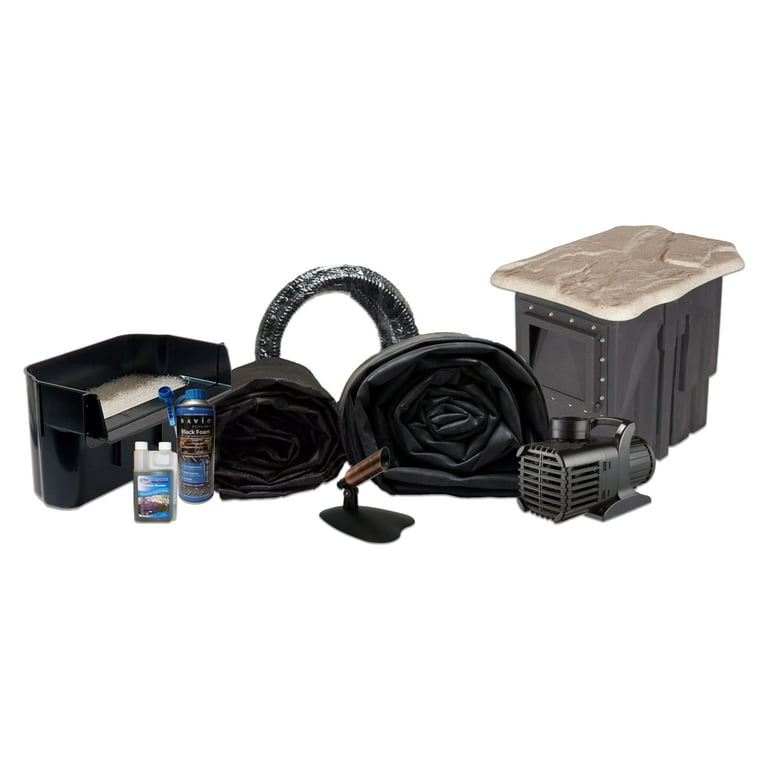The image showcases an assortment of automotive and camping accessories arranged haphazardly. Centered in the picture is a bottle of windshield wiper fluid and a bottle of foam sealant. To the left, a plastic container appears filled with white road salt. Dominating the background, two air mattresses are propped up, partially obscuring what looks like an engine air cleaner behind them. In the foreground, what resembles a microphone stand—potentially a jack handle—stands prominently. Nearby, an air pump is positioned in the front corner, adding to the clutter. A plastic storage tub with a white top, reinforced with several rivets for front access, completes the scene. The collection appears to be a mix of items useful for both car maintenance and outdoor adventures.